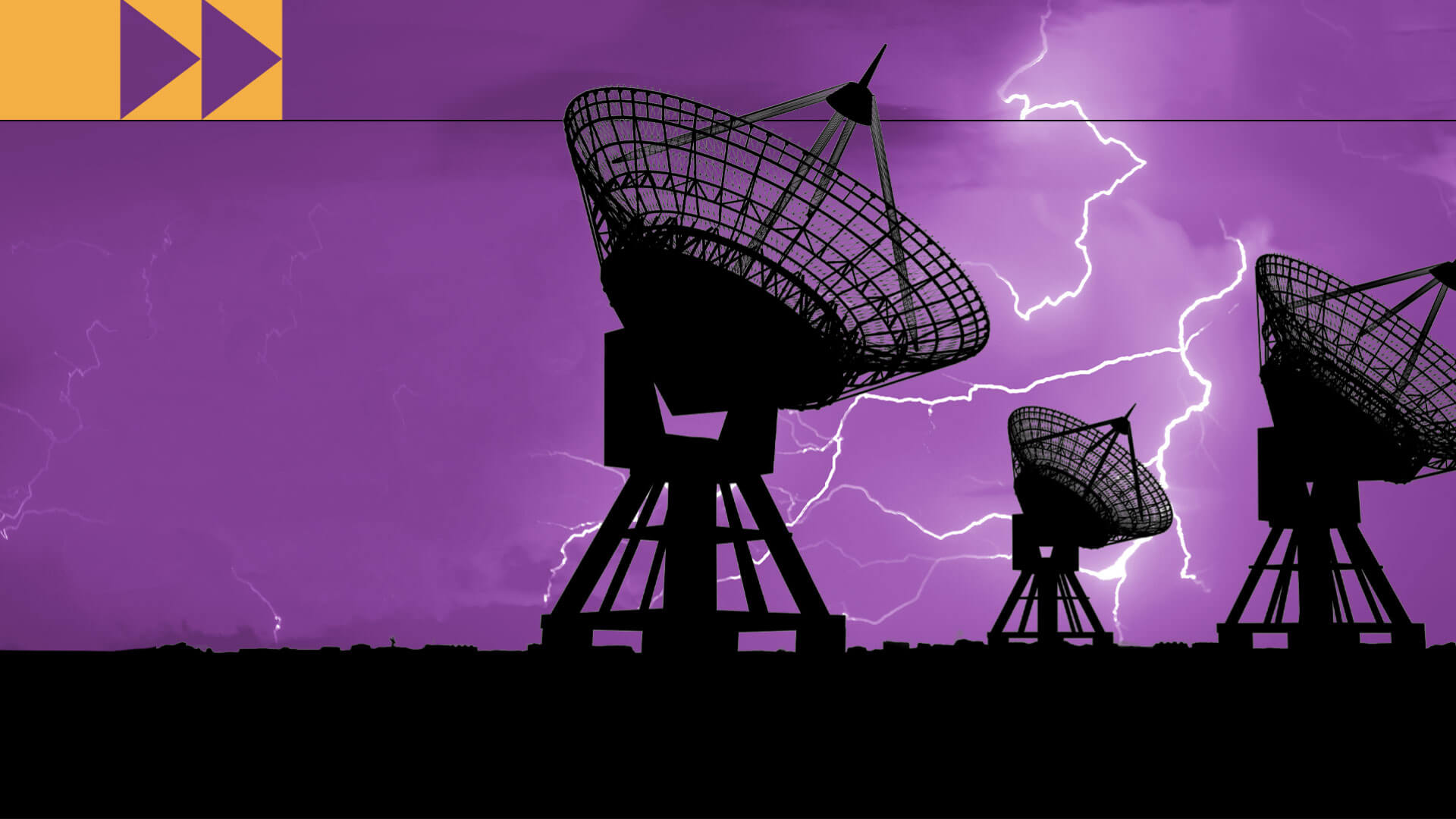The photograph features a striking contrast of dark silhouettes against a vivid purple sky. Dominating the scene are three large satellite dishes or radar structures with circular tops, each mounted on tripod-like stands and shadowed in pitch black. These dishes are pointing upwards and slightly to the right, seemingly attracting the five prominent lightning bolts that illuminate the sky in different shades of purple, with more intense brightness where the lightning strikes. In the distant background, low-lying buildings barely rise above the horizon, adding to the silhouetted landscape. The ground is completely black, merging seamlessly with the silhouetted structures. In the upper left corner of the photograph, a superimposed orange rectangle contains two purple triangles pointing to the right, resembling a fast-forward icon. The overall scene evokes a mysterious and electrifying atmosphere, accentuated by the dramatic interplay of light and dark.